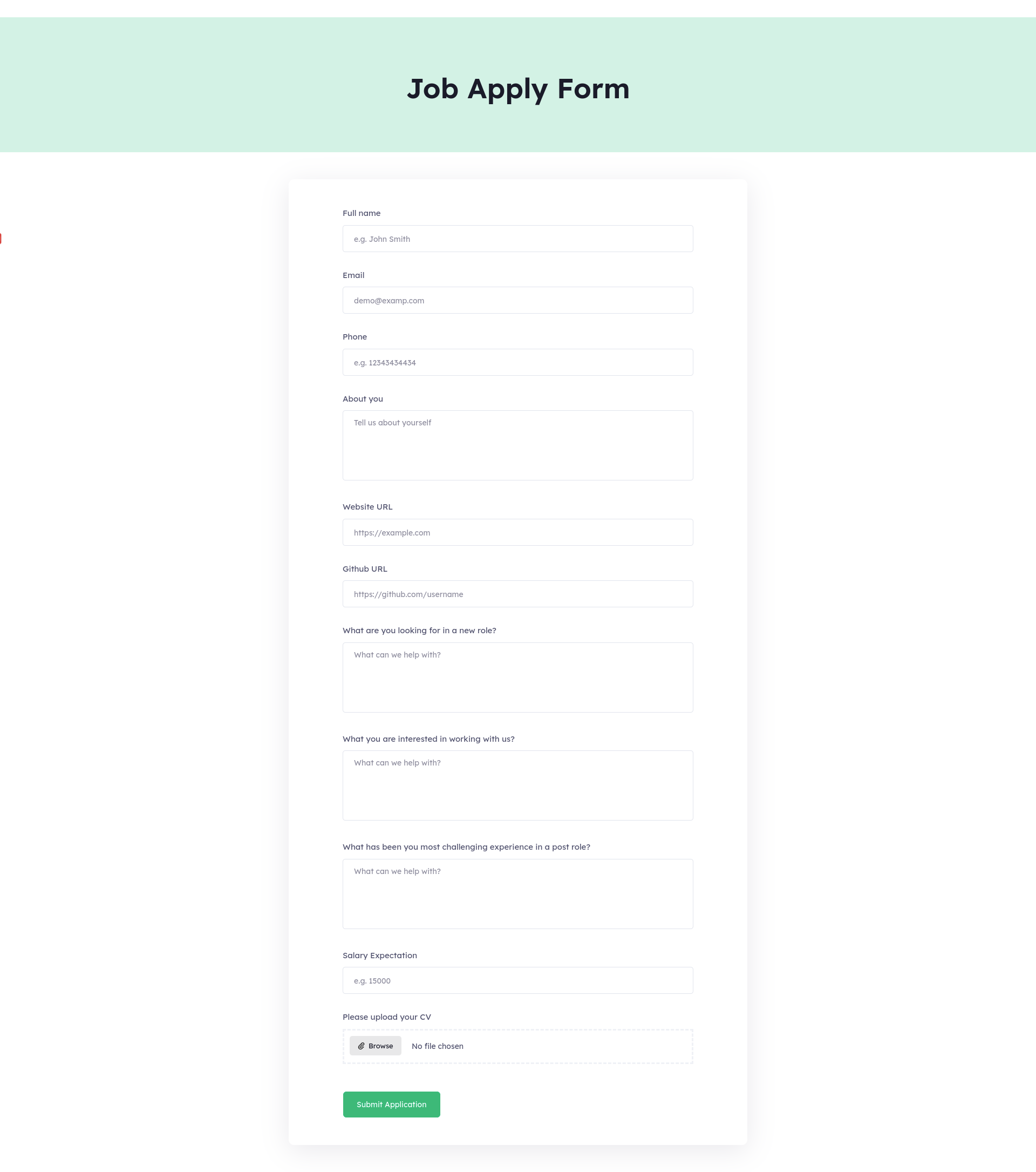The image is a screenshot of an online job application form. At the top of the form, there's a blue rectangular banner with the text "Job Apply Form" in black letters. The form contains several fields labeled as follows: "Full Name," "Email," "Phone," "About You," "Portfolio URL," and "LinkedIn URL." There is also a section labeled "What are you doing?" and "What are you looking for?" Near the end of the form, there's a designated area for uploading a resume. At the very bottom of the form, there's a small rectangular button in a greenish-blue color with the text "Submit." The overall design is minimalistic, primarily using black and white with no images, doodles, or additional colorful elements aside from the top banner and the submit button. The purpose of the various URL fields seems to be for applicants to provide links to their online portfolios or professional profiles.